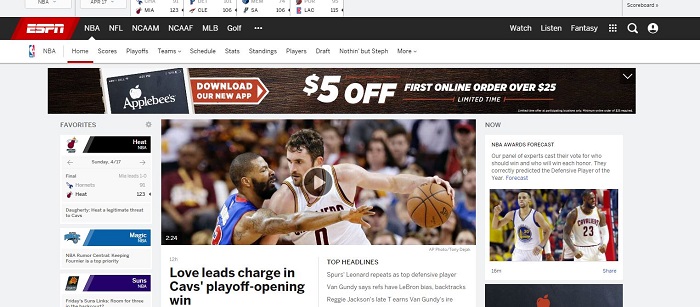This image captures the ESPN website in its entirety, showcasing a dynamic and content-rich interface. At the top of the page, the navigation bar prominently displays tabs for various sports categories, including NBA, NFL, NCAAM, NCAAF, MLB, and Golf, followed by a dropdown option indicated by an ellipsis. Positioned to the far left of these tabs are additional links for Watch, Listen, and Fantasy, aligned with icons for a three-by-three grid menu, search functionality, and user profile access.

Directly beneath the navigation bar is an elongated advertisement banner promoting an Applebee's special offer. The advertisement announces a 5% discount on first-time or online orders over $25, emphasizing the limited-time nature of the deal.

Continuing down the webpage, a variety of articles and multimedia content are displayed. Centrally located is a prominent video feature with a play button icon, inviting viewers to watch. The headline beneath this video highlights a significant sports event: "Love Leads Charge in Cavs Playoff Opening Win," encapsulating the Cavaliers' successful playoff opener led by a standout performance from a player named Love.